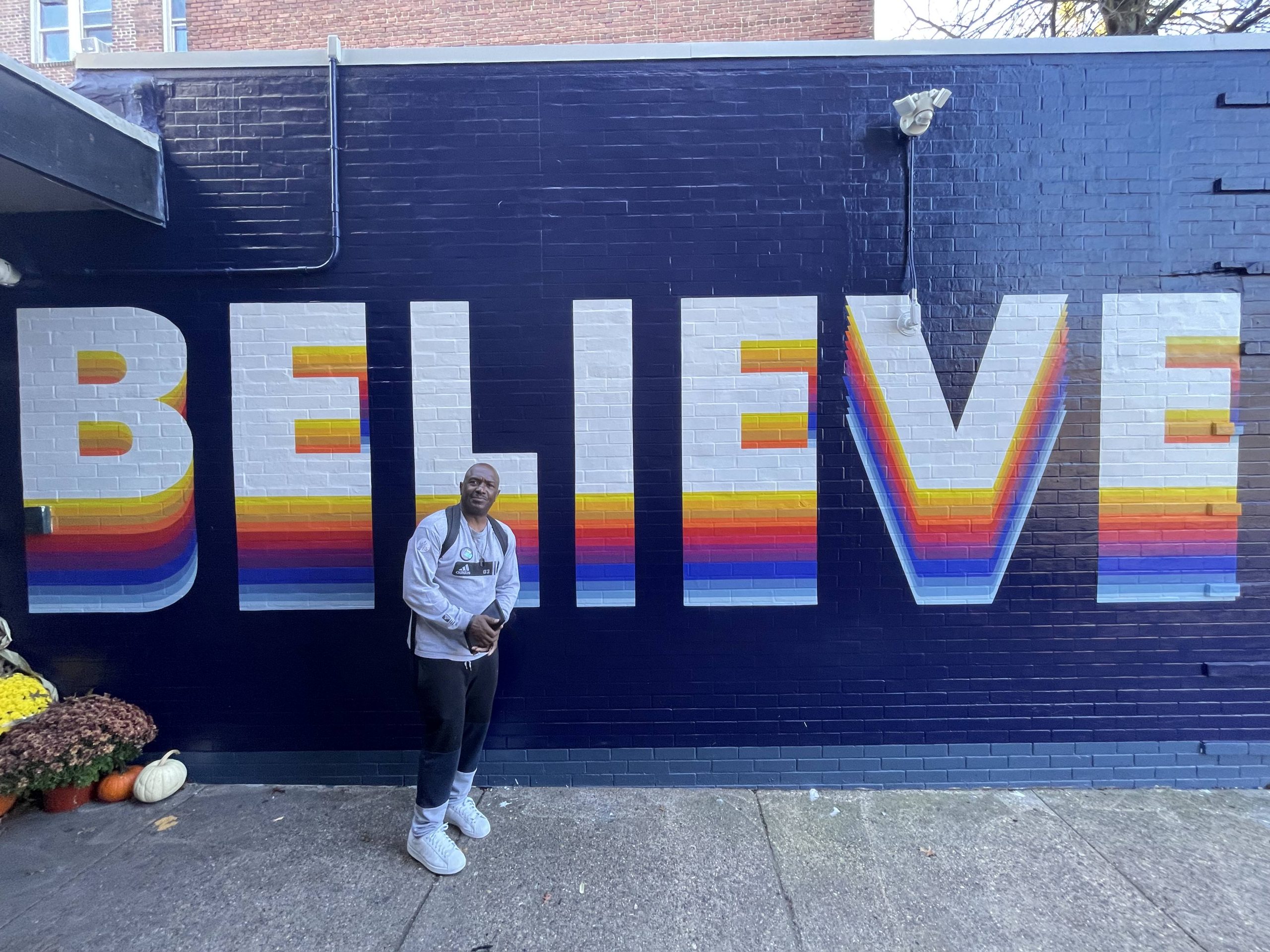In the photograph, a man stands against a dark navy blue brick wall that features a striking mural of the word "BELIEVE" painted in prominent white letters. Below the white text, a multicolored, 3D drop shadow effect adds depth with layers transitioning through yellow, orange, red, and various shades of blue, ending in a light blue almost white hue. The man, who appears to be Black, is dressed in a long-sleeved gray Adidas shirt with black trim, black sweatpants with white trim at the bottom, and white sneakers. He has a backpack on his back and holds what seems to be a tablet in his hand. To the left of the man, in the corner of the image, there are several plants in pots, including flowers and two pumpkins—one orange and one white—adding a touch of natural color to the scene. The arrangement of the man and the word "BELIEVE" on the wall is centrally focused, making it the visual anchor of the photograph.